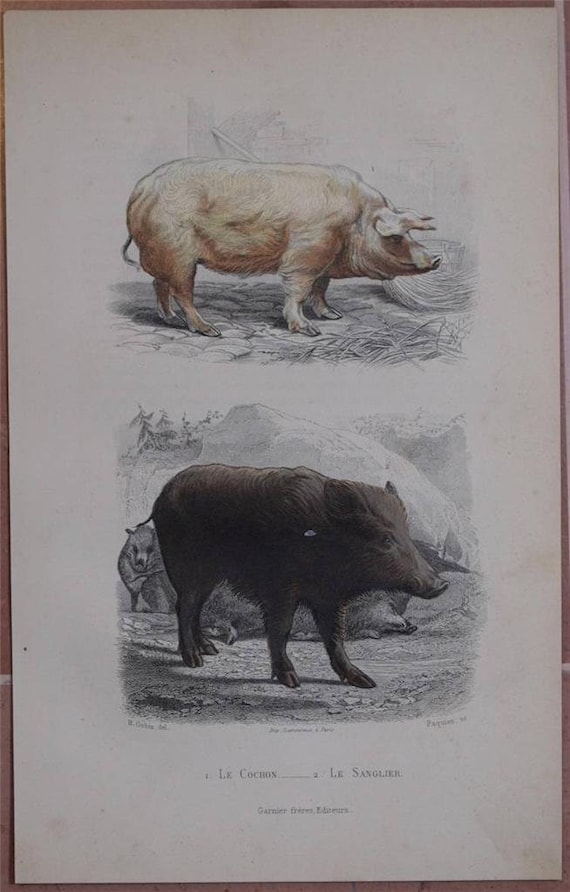This detailed illustrative poster features two distinct pig-like animals rendered with colored pencils. In a portrait-oriented layout, the top part of the poster showcases a modern-day pig in pinkish-orange hues standing alone on a grayish ground. Below it, a darker, wild boar—or possibly a warthog—is depicted, characterized by longer legs, a longer snout, and shorter ears, blending earthy browns with the gray floor beneath it. Surrounding this central imagery is a narrow brown border. The background of the illustrations appears brownish, providing a subtle contrast to the gray ground where the animals stand. Accompanying the illustrations is text in black and white, positioned at the bottom of the poster. The text reads "Les Cochons, Les Sangliers," indicating in French, "The Pigs, The Boars."